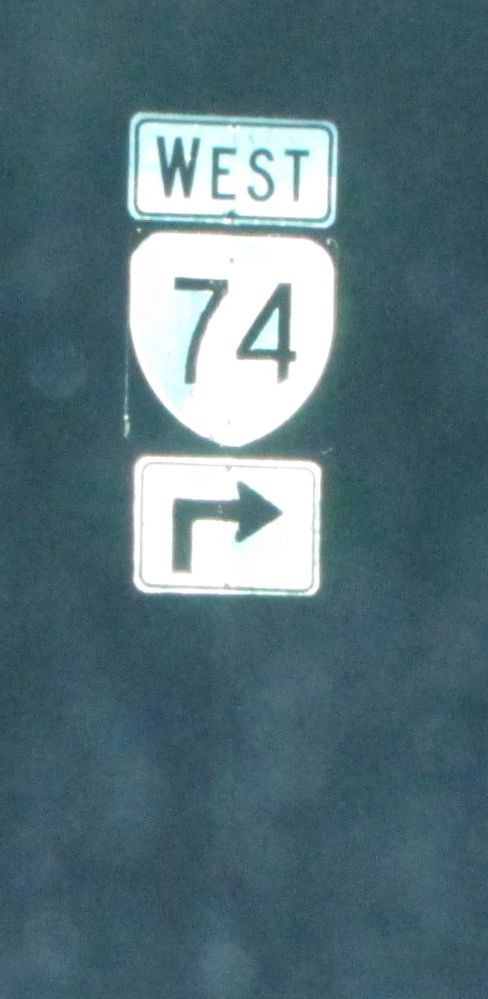A series of three street signs are prominently displayed against a dark, cloudy gray background, though they appear to be illuminated by sunlight. The top sign is a white rectangle with a black border, boldly displaying the word "West" in black letters. Below it, there is a state route sign, also white, featuring the number "74" in black. The bottom sign is another rectangular white sign with a black border, featuring an arrow that indicates a sharp right turn. The overall message indicates an upcoming right turn to continue west on Route 74. Despite the background not being part of the scene, the signs are distinct and brightly lit.